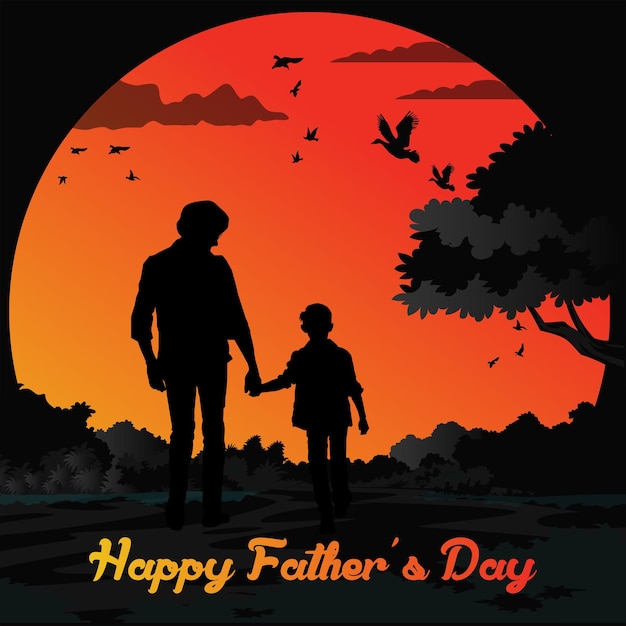The image is a digital rendering commemorating Father's Day, likely designed for a card. The prominent text at the bottom reads "Happy Father's Day," with the words transitioning in color from yellow to light orange and finally to a dark sunset orange. The main visual shows a silhouette of a father and son walking hand in hand into the distance, depicted as black shadows against a vivid background. 

The father is dressed in a cuffed dress shirt and regular pants, with something sticking out of his pocket, mirroring the son's similar attire. This "like father, like son" theme is emphasized by their identical clothing. The scene is set in an open field at sunset, with the large circular sun dominating the background and casting a warm, gradient glow from yellow to red-green hues across the sky.

Birds flying in the distance add to the tranquil ambiance, while a standard oak tree with abundant leaves juts out from the right edge of the image. Fainter shadows of additional trees and bushes can be seen in the background. The entire composition is rendered in a silhouette style, with the sun, birds, and a few light gray clouds providing the only variations in color against the otherwise black shadowy figures and landscapes.